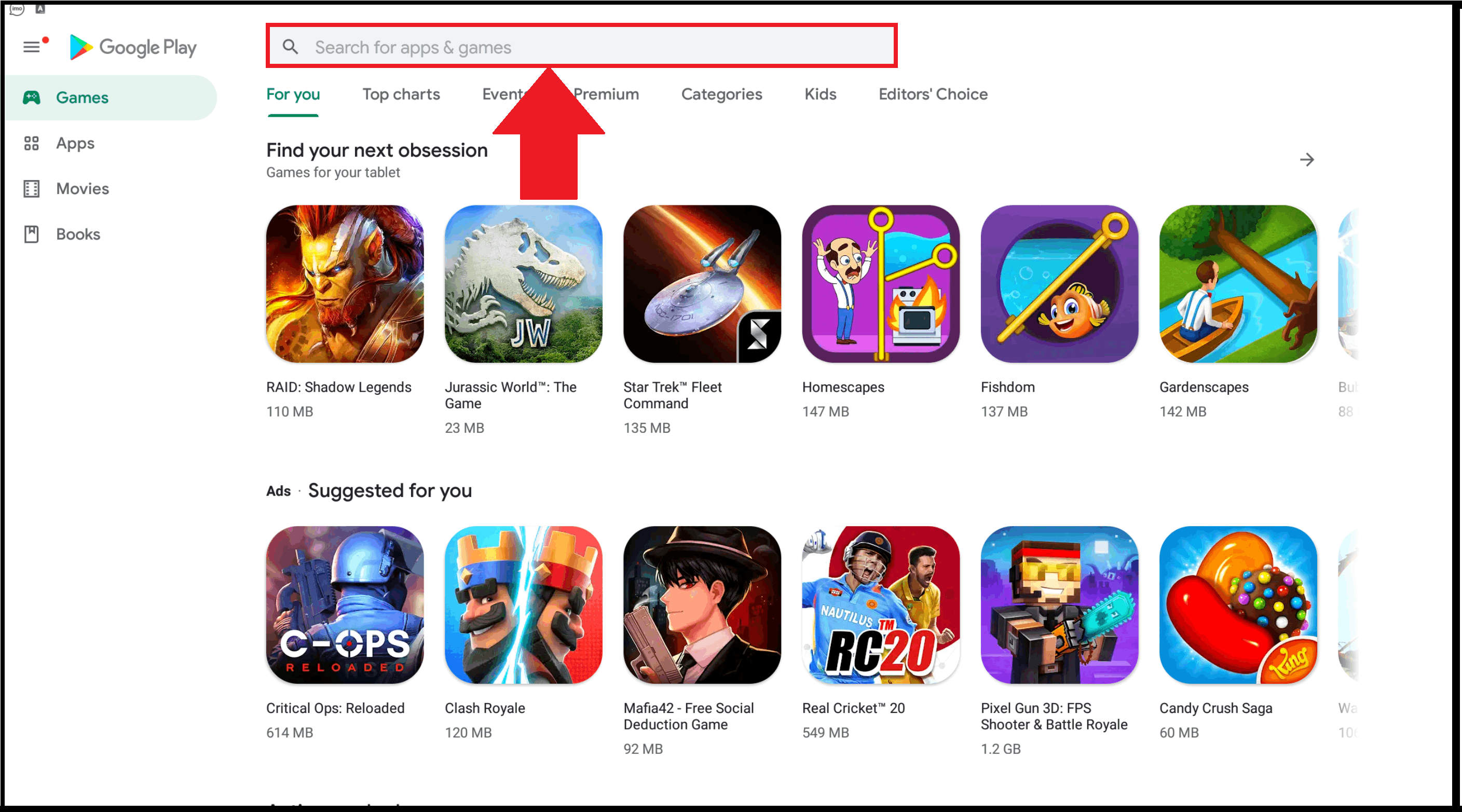This screenshot showcases the Google Play Store, specifically under the "For You" tab within the Games section. A prominent red bar and an arrow highlight the search bar for apps and games, providing guidance for new users on how to locate desired games. The interface reveals several selectable tabs including "Top Charts," "Events," "Premium," "Categories," "Kids," and "Editor's Choice" to explore different types of content. In addition to games, other sections accessible from the Play Store include apps, movies, and books.

Within the Games section, around 12 games are prominently displayed as recommendations, featuring titles such as "Raid: Shadow Legends" (noting a download size of 110 MB), "Jurassic World: The Game," "Star Trek: Fleet Command," "Homescapes," "Fishdom," "Gardenscapes," "Critical Ops: Reloaded," and "Clash Royale," among others. This screenshot serves as an instructional tool for beginners, illustrating how to navigate the Play Store and discover various entertainment options.